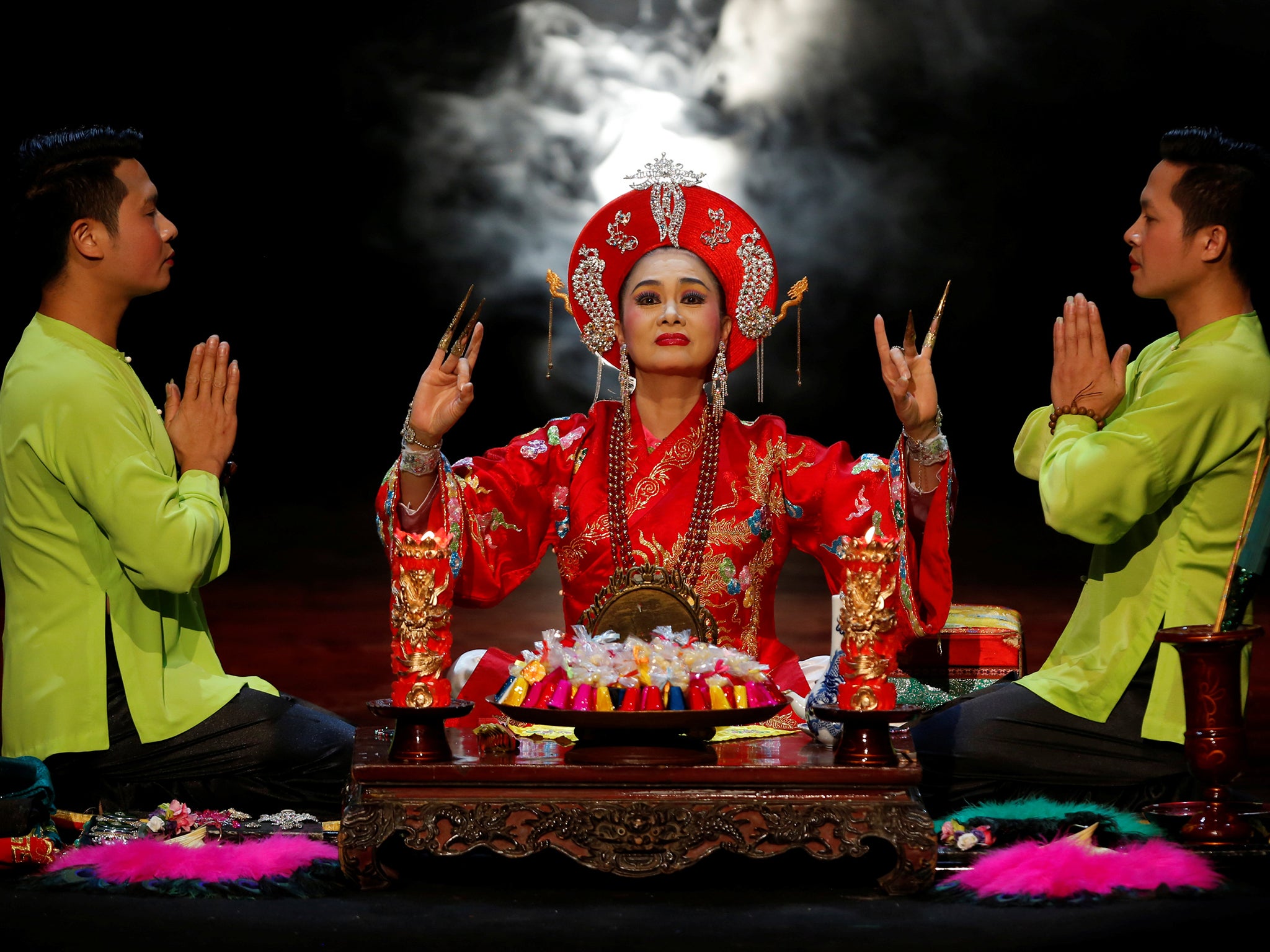In the center of a visually striking photograph, an Asian woman is dressed in an elaborate red silk robe adorned with intricate gold, blue, and white floral designs. Her dramatic outfit is complemented by a regal red hat with diamond-like designs, resembling a crown, which partially covers her face. She holds her hands aloft, revealing long, sharp spikes protruding from her pinky fingers, a traditional element suggesting cultural significance.

On either side of her, two men with dark brown skin and black hair sit kneeling on cushions, their eyes closed in what appears to be a gesture of prayer or respect. Both men are wearing identical lime green pullover shirts and black pants, with their hands clasped together in front of their faces.

In front of the woman, there is a small, polished wooden box with a glossy black tray filled with colorful spools of thread in pink, yellow, blue, and orange. Alongside these items are two circular stands topped with cylinders featuring red and gold designs. The background is predominantly black, dramatically illuminated by wisps of white smoke emanating from behind the woman's head, adding an ethereal quality to the scene, which seems to be a ceremonial ritual captured in vibrant detail.